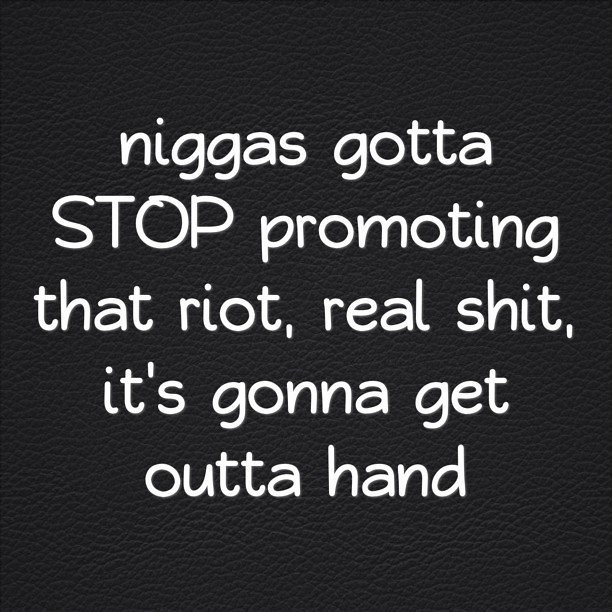The image displays a black poster board with white text, formatted in a square shape with multiple horizontal rows. The message, conveyed entirely in lowercase except for the capitalized word "STOP," reads: "niggas gotta stop promoting that riot, real shit, it's gonna get out of hand." Commas follow the words "riot" and "shit," with no period concluding the statement. The poster emphasizes a warning about promoting riots. This stark and simplistic design uses no other colors or images, focusing solely on the textual warning and the black-and-white contrast.